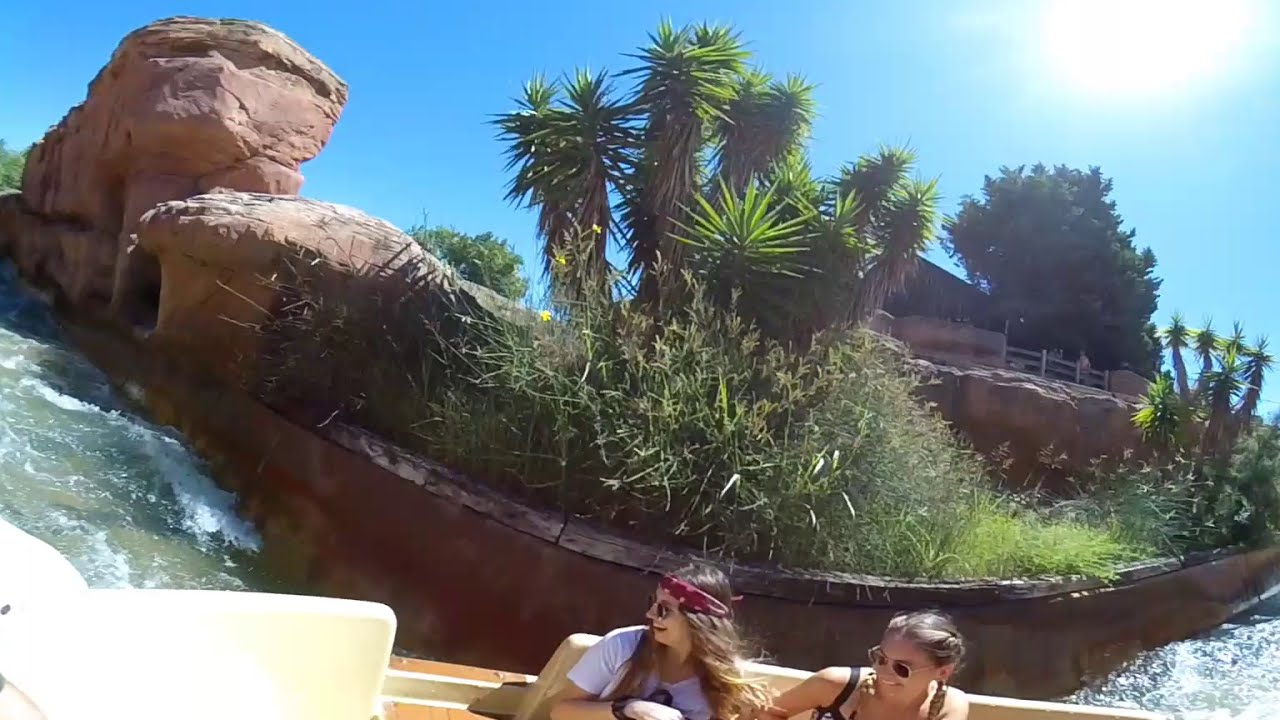In the bottom center of the image, two women wearing sunglasses are sitting in a wooden canoe or boat on what appears to be a man-made lazy river. The woman on the left has long hair adorned with a purple headband, while the woman on the right has her hair in braids. Surrounding them is a scenic backdrop, featuring a curved brown barrier separating them from a lush garden of tropical trees, taller leafy trees, various plants, and grass. To the upper left, there are clay or adobe rock formations with what looks like an entrance. The sky above is bright blue and cloudless, with the sun visible in the upper right-hand corner, casting a warm glow over the scene.